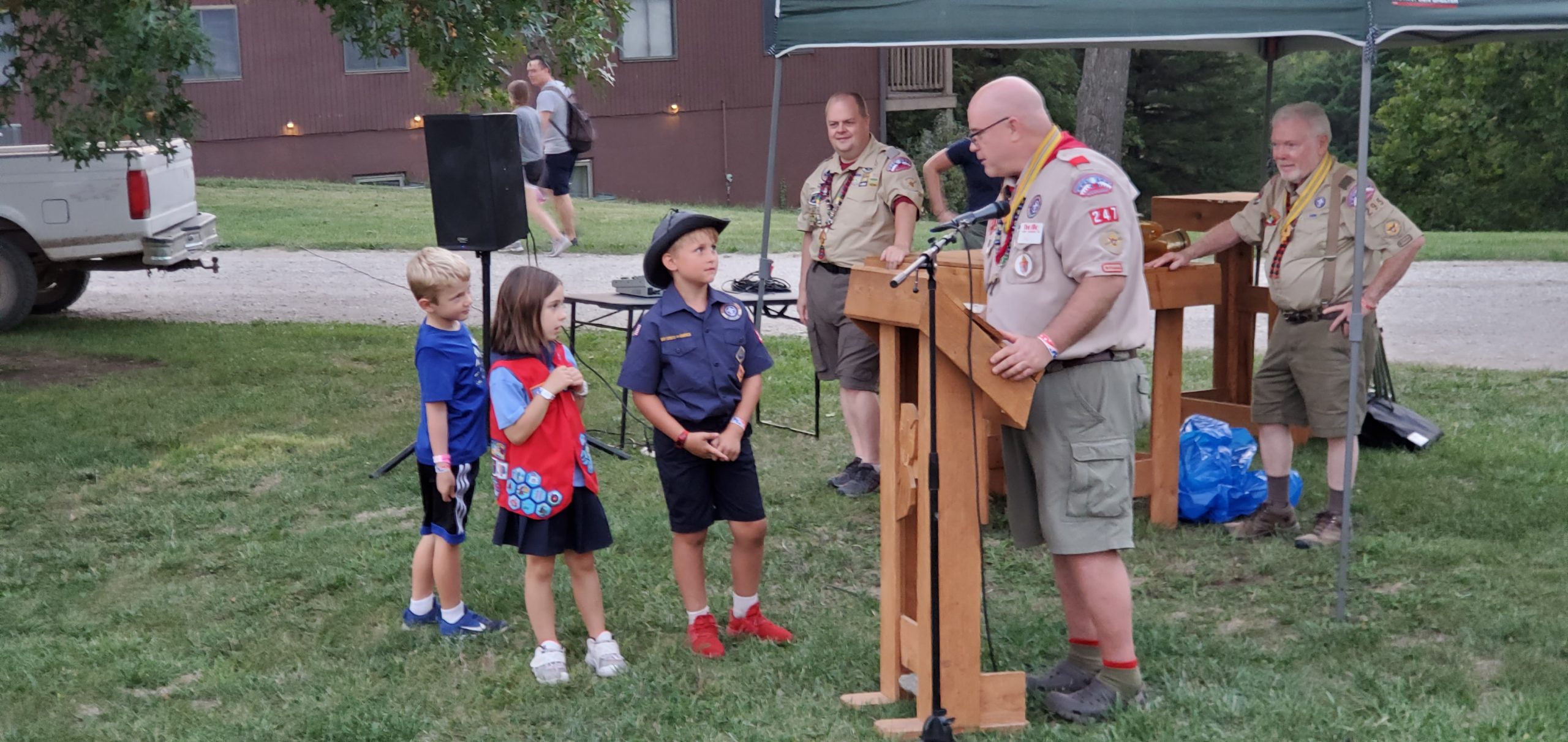In this image, a Boy Scout leader is seen standing at a wooden podium, speaking into a microphone. He is dressed in a tan Boy Scout uniform adorned with various badges and patches. Behind him stand two other Scout leaders, similarly uniformed in tan shirts and cargo shorts, under the shade of a green tent. To the right of the podium, three children listen attentively. One boy, directly facing the speaker, wears a blue short-sleeved button-down shirt embellished with badges, blue shorts, red shoes, and a hat. Beside him stands a girl in a red vest with patches, and behind her is another boy in a blue t-shirt and black and white shorts. The grassy background reveals the rear end of a white pickup truck on the left, a dirt or gravel walkway, and an outline of a dark purple or brown building with windows. Tall green trees fill the upper right corner of the image, completing the scene.